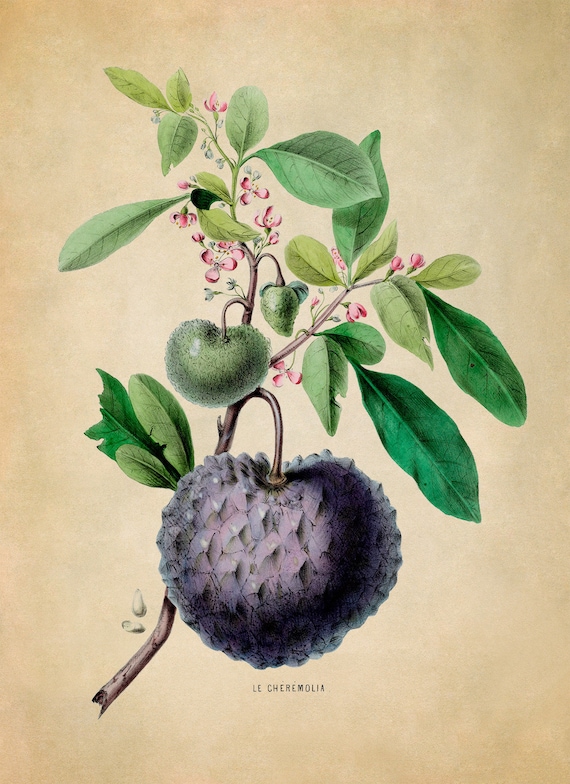This tall, vintage botanical print, set against a tan-ish white background that is darker in the corners and lighter in the middle, showcases a detailed illustration of a plant named "Le Caramolia," as labeled in black, all caps text at the bottom. The plant features a slender, dark brown stem branching out into green shoots with freshly grown leaves. From the branches, delicate pink flower buds bloom, clustering in multiple areas. Prominently depicted are the plant's fruits: an unripened green fruit and a larger, textured, plum-like purple fruit that has a jagged appearance. Both the leaves, characterized by their varying shades of green, and the vibrant flowers, contribute to the scientific representation of this botanical specimen, emphasizing its intricate natural beauty.